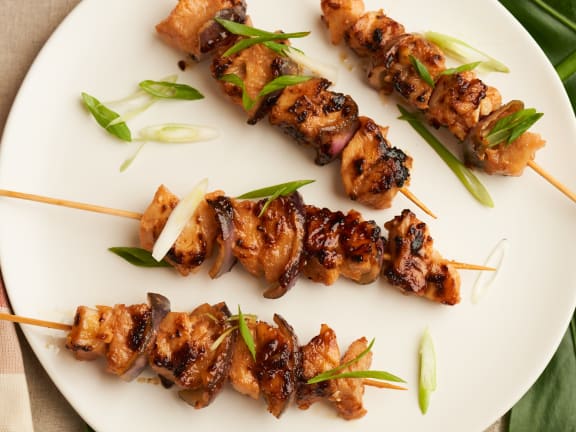This image showcases a large white plate set against a subtly obscured background. Surrounding the plate are faint hints of greenery, possibly foliage, and a brown area on the left suggesting a table surface. The plate prominently features four dainty meat skewers, composed of grilled chicken pieces. Garnishing the skewers are sprigs of rosemary, their pointed leaves adding a touch of visual appeal. Notably, the second skewer holds a delicate white petal, likely from a chrysanthemum, enhancing the presentation with a floral accent. The skewers, despite their delicate size, are arranged meticulously, creating an inviting and appetizing display.